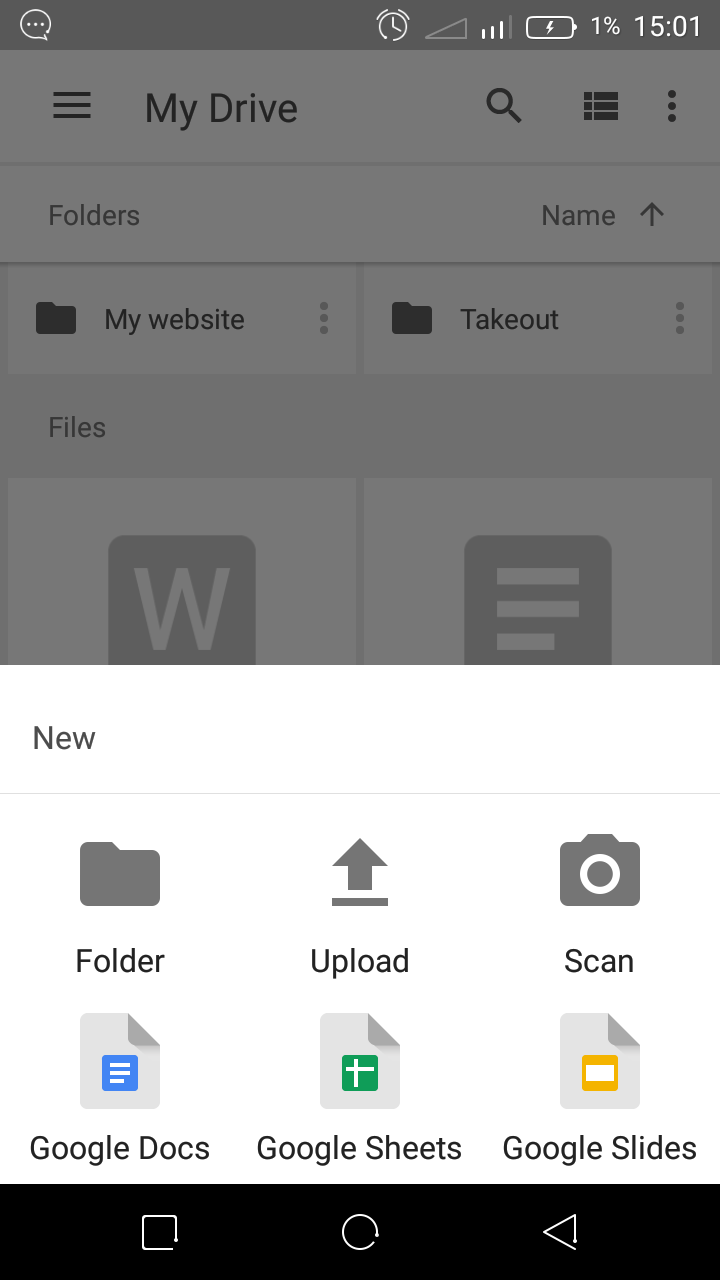In this image, a smartphone screen displays the Google Drive interface. At the top of the screen, the "My Drive" section is visible against a slightly transparent white background. Below "My Drive," there are various folders and files. Specifically, two folders are prominently shown: "My Website" on the left and "Takeout" on the right. 

Further down, partially obscured by a pop-up menu at the bottom, are some files. One file features an icon with a white "W" on it, indicating it might be a Word document. The overall background of the main page is a clean white, providing a clear view of the contents.

At the bottom of the image, a pop-up menu titled "New" is displayed, indicating options for creating new items. This menu lists six options: "Folder," "Upload," and "Scan" at the top, all depicted in grey. Below these, three more options rendered in light grey are shown with corresponding document icons: "Google Docs" in blue, "Google Sheets" in green, and "Google Slides" in orange and white. This tidy, detailed layout emphasizes efficiency and easy navigation within Google Drive on a smartphone interface.